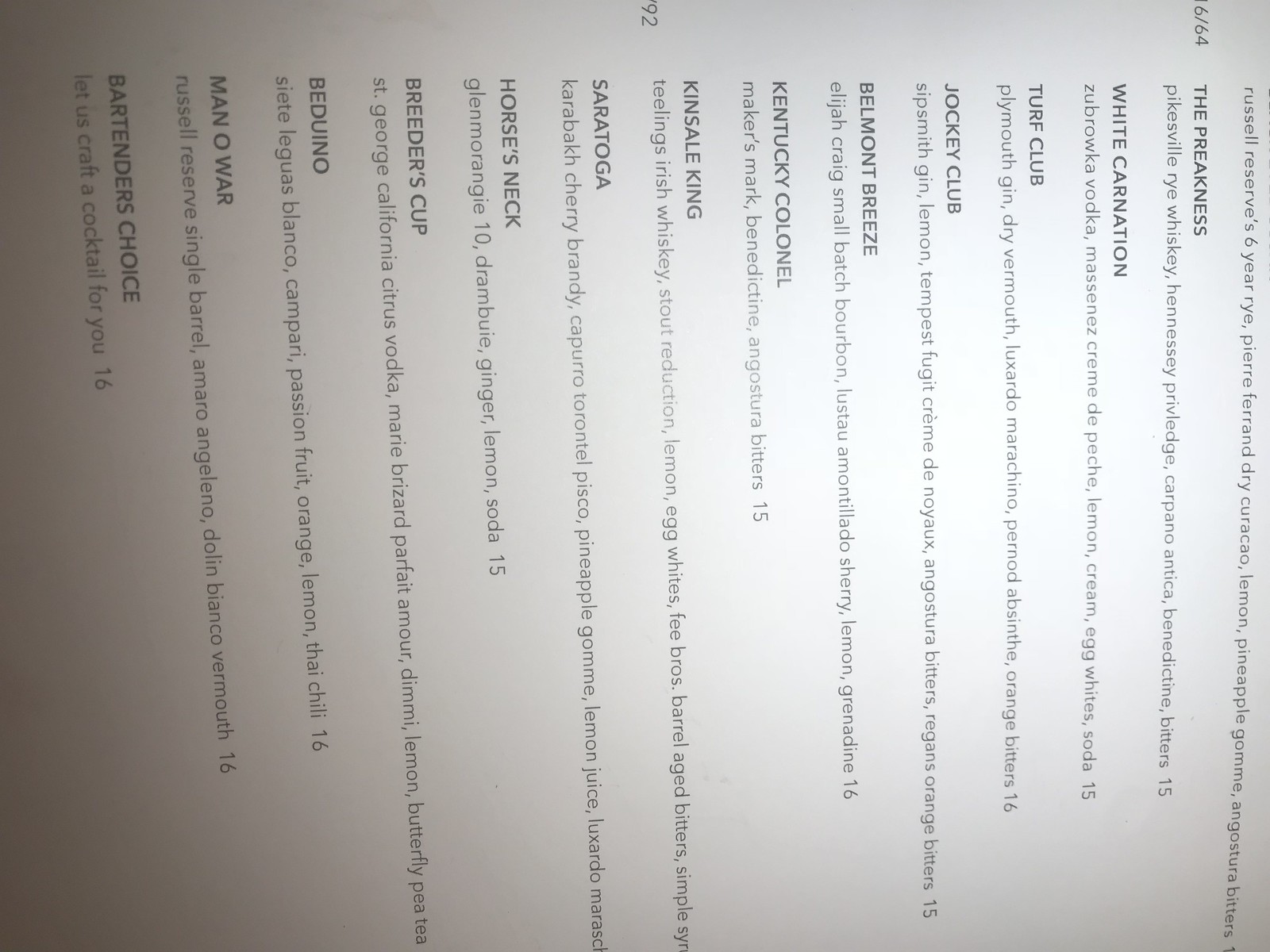A drinks menu displayed on its side features a collection of creatively named cocktails, each with a detailed list of ingredients. The menu has black text set against a white background. Among the drinks listed are:

- The Preakness: A potent blend of Plain Pikesville Rye Whiskey, Hennessy Privilege, Carpano Antica, Benedictine, and Bitters.
- White Carnation
- Turf Club
- Jockey Club
- Belmont Breeze: Crafted with Elijah Craig Small Batch Bourbon, Listel Amontillado Sherry, Lemon, and Grenadine.
- Kentucky Colonel
- Kinsdale King
- Saratoga
- Horse's Neck
- Breeders' Cup
- Beduino
- Man O' War
- Bartender's Choice: Likely a creation of the bartender's choosing, tailored to the patrons' preferences.

The diverse array of drinks pays homage to names associated with prestigious horse-racing events and figures, hinting at a theme of tradition and sophistication. The Belmont Breeze's inclusion of Amontillado Sherry brings a hint of mystery and intrigue, while the Preakness offers an intense experience with its robust combination of spirits.